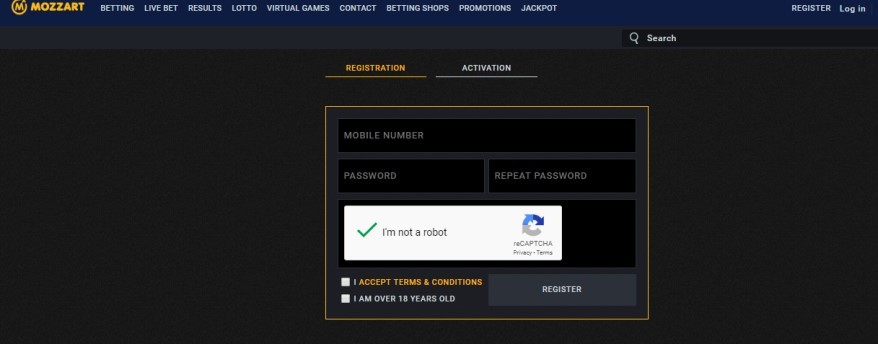This screenshot captures the interface of the Mazart betting and lottery platform. At the very top of the interface, the Mazart logo is prominently displayed next to a navigation bar featuring several options: Betting, Live Bet, Results, Lotto, Virtual Games, Contact, Betting Shops, Promotions, and Jackpot. In the top right-hand corner, there are buttons for 'Register' and 'Log In', with a search bar located just below these buttons.

The main section of the interface showcases two tabs - one for Registration and one for Activation. The Registration tab is highlighted in orange, indicating that it is currently active. Within this tab, users can enter their mobile number, create and confirm a password, and complete a reCAPTCHA test to verify they are not a robot. Additionally, there are two checkboxes: one in orange text for accepting the terms and conditions, and another in white text affirming that the user is over 18 years old. To the right of these input fields, there is a gray 'Register' button ready for users to finalize their registration.

The overall design is clean and user-friendly, ensuring that new users can easily navigate and complete the registration process.